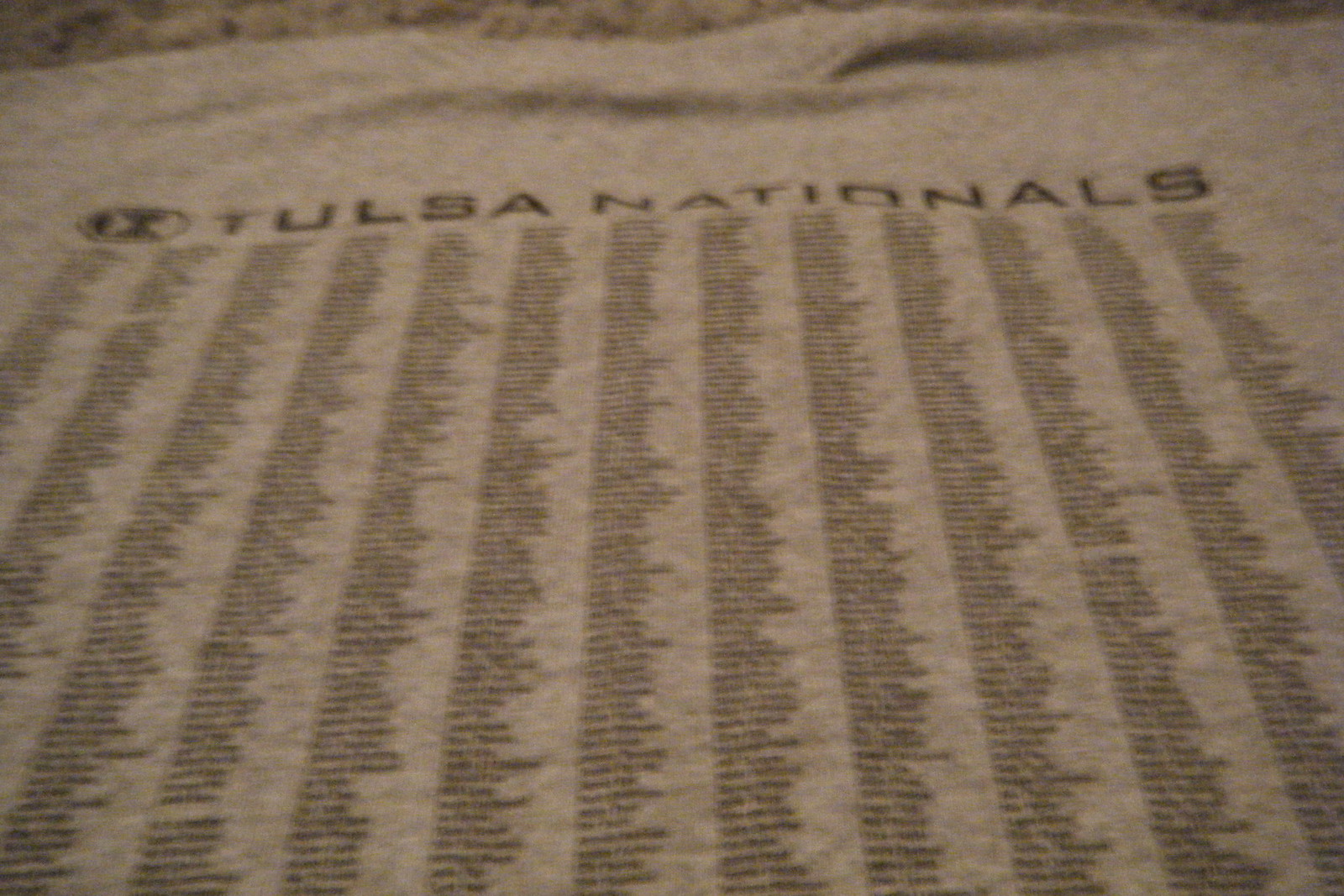A light gray cotton t-shirt is neatly laid flat, occupying the entire frame of the image. The back of the shirt prominently displays the text "Tulsa Nationals" in bold black ink at the top. Beneath this title, there are 13 columns filled with names, but they are too small and blurred to be legible. The t-shirt's surface is smooth, suggesting it may be resting on a bed. In the top right-hand corner of the image, a small portion of a different fabric is visible, potentially from a chair or sofa.